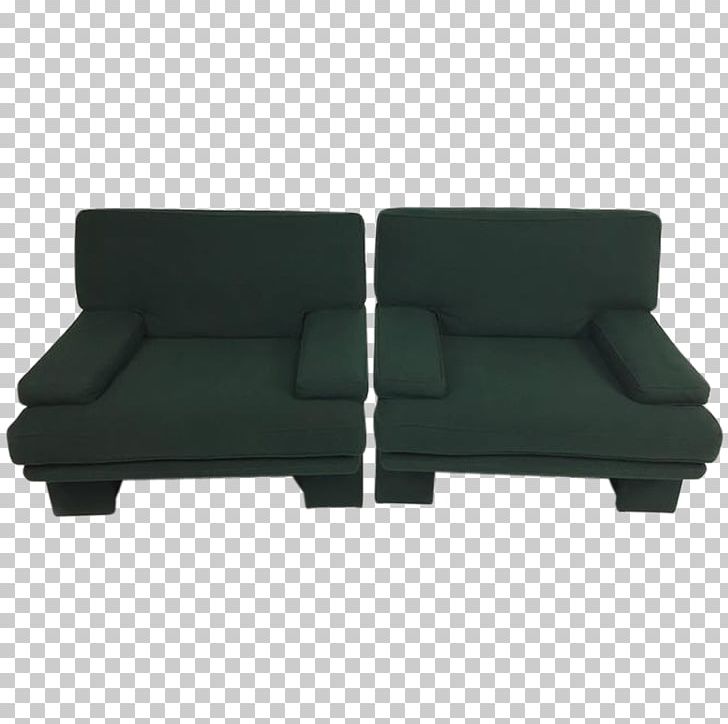The image portrays a close-up shot, likely captured from a graphic design program, suggested by the gray and white checkered background commonly used to indicate transparency in software like Photoshop. Centrally positioned are two identical dark green chairs, closely aligned side-by-side. Each chair is upholstered in a fabric material, exhibiting a boxy and squat shape that appears to be comfortable. They feature two large armrests on either side of the wide seat, a low backrest, and are supported by four short black legs, possibly made of wood. The chairs, which resemble a forest or olive green shade, show no signs of wear, tears, or stains, implying they are in pristine condition. The overall setup and presentation of the chairs evoke a polished and ready-for-advertisement feel, such as for a furniture catalog or magazine.